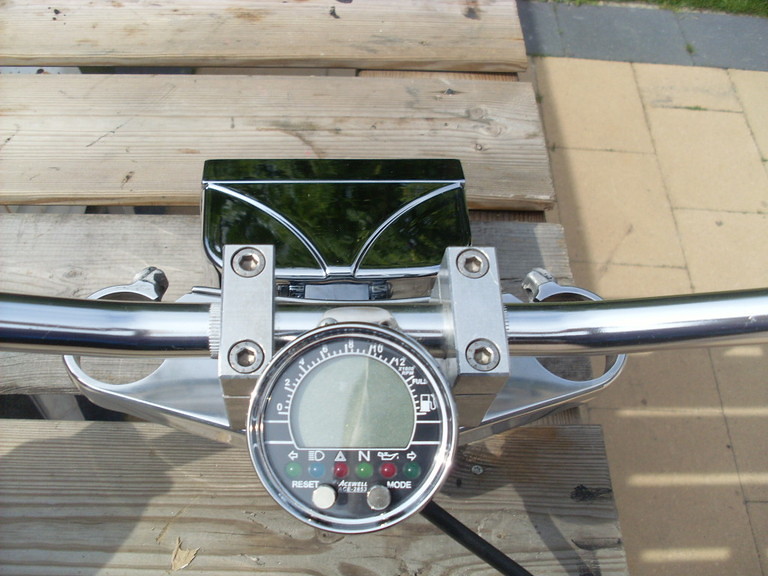This is an image of a bike's odometer or dashboard gauge. At the bottom center of the picture is a silver, circular metal device. The interior of the circle is predominantly black, featuring an LCD screen in the middle, which appears to be turned off and thus displays a gray color. Surrounding the top half of this circular face are white lines and numbers indicating measurements from 0, 2, 4, 6, 8, 10, 12, up to 'Full,' accompanied by an icon of a gas tank.

In the lower portion of the circle, there are several symbols each accompanied by different colored lights: a left arrow with a green light, an indistinguishable symbol with a blue light, a triangle with a red light, a letter 'N' with a green light, a symbol resembling a genie lamp with a red light, and a right arrow with a green light. At the very bottom of the circle, there are two buttons labeled 'Reset' on the left and 'Mode' on the right.

Above the circular device, silver handlebars extend horizontally. The entire setup is mounted on what appears to be a plank of wood.